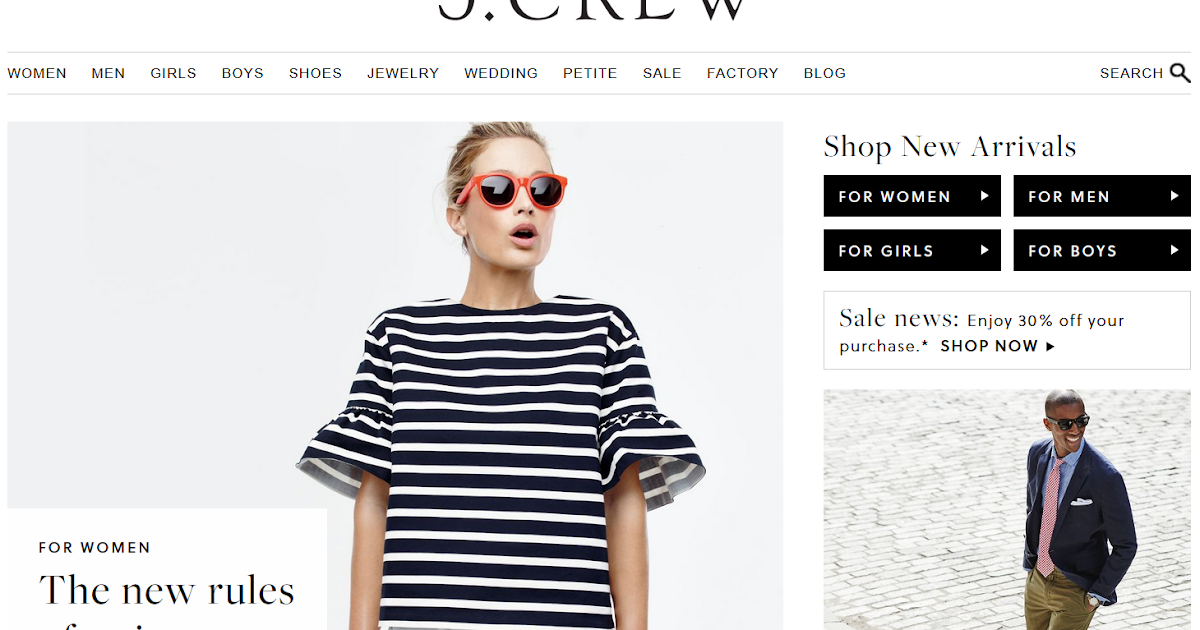This is a screenshot of the J.Crew website, showcasing its header and promotional images. At the top, partially cut off, are the brand's name in bold black letters: "J.CREW". Below this header, a navigation menu offers various category options: Women, Men, Girls, Boys, Shoes, Jewelry, Wedding, Petite, Sale, Factory, and Blog. A black magnifying glass icon appears next to the word "Search", indicating a search feature.

The central image features a fair-skinned woman with blonde, slicked-back hair, wearing red-framed sunglasses. Her mouth is open, and she is dressed in a top with black and white horizontal stripes. The top has quarter-length sleeves with ruffled ends. To her left, text reads: "For Women, The New Rules". To her right, promotional text states: "Shop New Arrivals for Women, for Men, for Girls, for Boys. Sale News: Enjoy 30% off your purchase. Shop now."

Below this, another photograph depicts a young African-American man standing on a white brick walkway. He is looking to the right with a big smile on his face. His close-cropped hair complements his stylish outfit, which consists of a blue blazer over a blue button-down collared shirt, a red necktie, and brown pants. His left hand is in his pocket, revealing a gold wristwatch on his wrist.